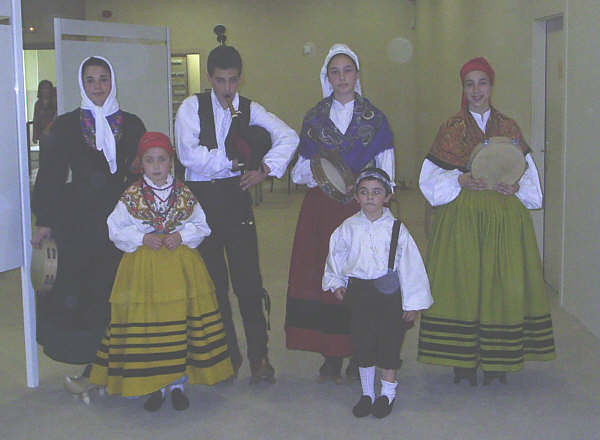In the image, a vibrant family, dressed in elaborate, colorful cultural outfits, is poised to put on a lively performance, evocative of a Mariachi band. The group includes both adults and children, with the adults appearing to be in their early twenties and the children significantly younger. The women wear long, ornate dresses in hues of red, green, and yellow, along with headbands and headdresses. The young boys are donned in smart suits, while a little girl stands out in a beautiful mustard-colored skirt paired with a red bandana. They are equipped with various musical instruments, with one man notably playing the bagpipes, and others holding tambourines. Their bright ensembles, including black shoes and detailed accessories, contrast vividly against the yellow walls and white doors of their home. Smiling broadly, they are ready to deliver an energetic and culturally rich performance.